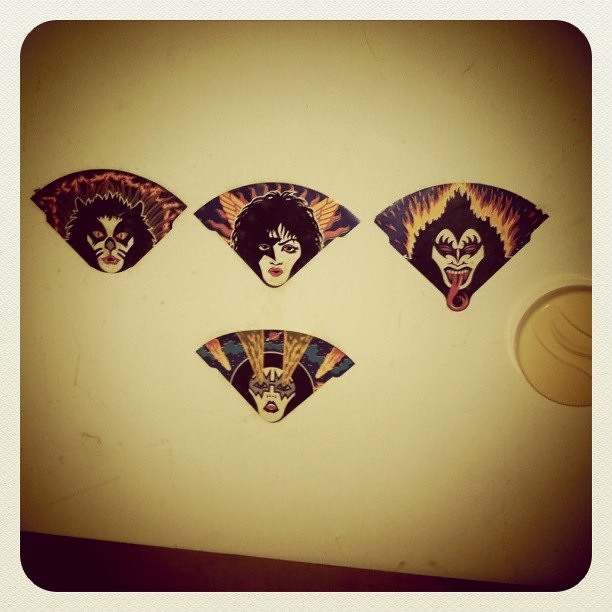The image is a slightly taller-than-wide photograph encased in a tan border. At its center lies an off-white wall, highlighted by a spotlight that cuts through the otherwise dark room. Mounted on this wall are four distinctive hand fans, each showcasing the face of a member of the band KISS, mimicking their iconic makeup designs. From left to right, the top row features a fan adorned with the face painted like a cat: white base, black eyes with whiskers, and red lips. Next to it is a fan of a white-faced man with a black star over his right eye (left to the viewer), shaggy black hair, and red lips. The third fan on the top showcases Gene Simmons, easily recognizable by his black hair, swirling tongue, and bat-like black eye makeup on a white face. Below these, in the bottom center, is a slightly smaller fan bearing the face with bat-styled makeup around the eyes, a white base, and red lips. On the right side of the image and partially cut off is a circular stick-on air freshener, described as similar to a Glade plug-in. The imagery of the fans blends a cartoonish style with dramatic, theatrical makeup reminiscent of the band's signature looks.